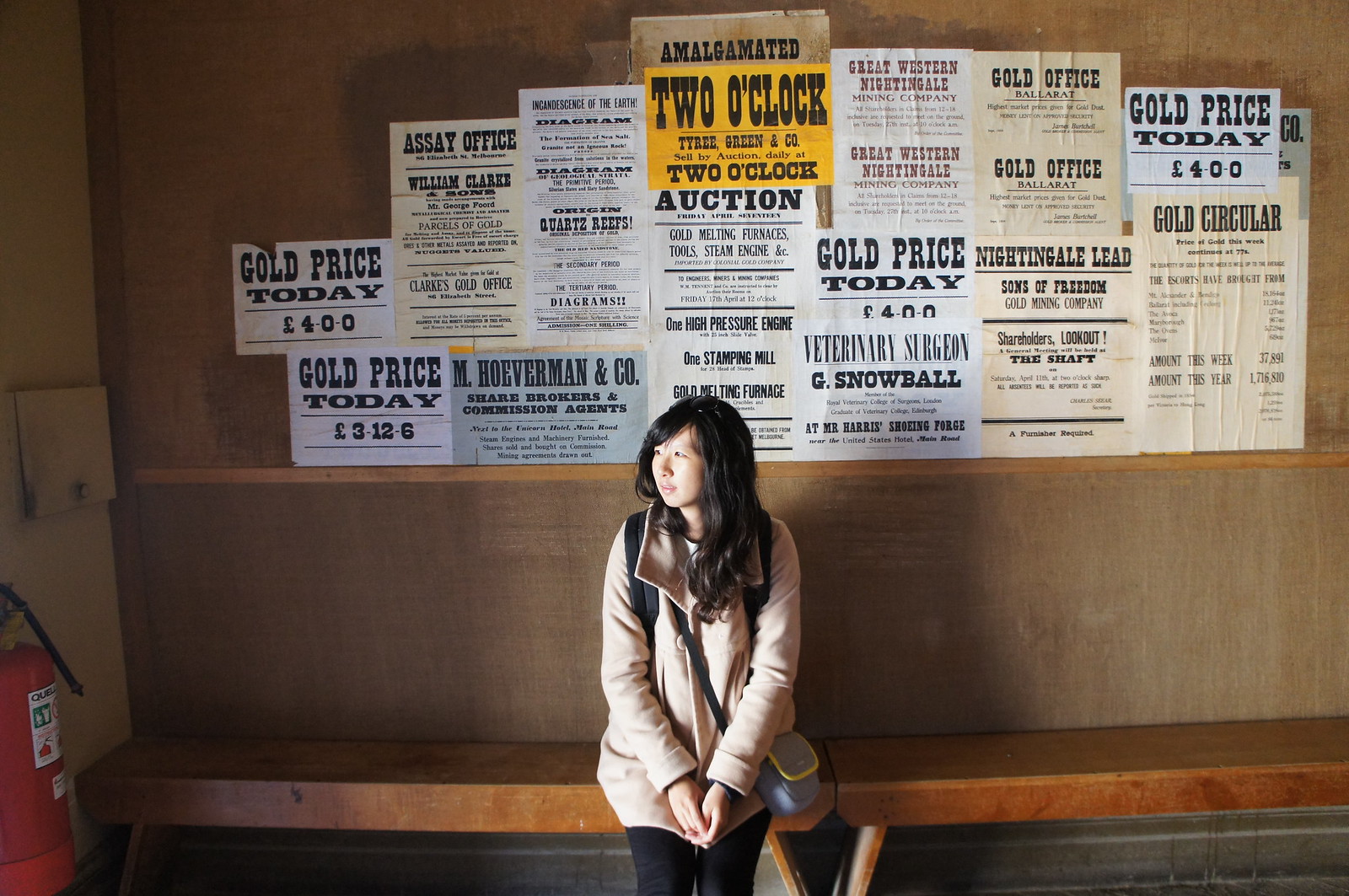This photograph showcases a young Asian woman seated on a wooden bench composed of two sections placed side by side to form a single long seat. She is wearing a light brown jacket and black pants. Her attire is complemented by a black backpack slung across her shoulder and a blue, yellow, and black purse diagonally strapped across her chest. The woman, with long dark hair, gazes thoughtfully toward the right side of the frame.

The setting appears to be an indoor room with large walls adorned with numerous posters and printouts featuring a variety of fonts and colors, predominantly black and white with some patches of orange, blue, and tan. Among these, text highlights include mentions of "Tyree Green and Company sell by auction daily at 2 o'clock," "Gold Office, Ballarat, highest market prices given for gold dust," and "Veterinary Surgeon G. Snowball at Mr. Harris's Shoeing Forge." Additionally, a yellow poster is notably present among the monochrome prints. To the left side of the image, part of a fire extinguisher can be seen mounted on the wall.